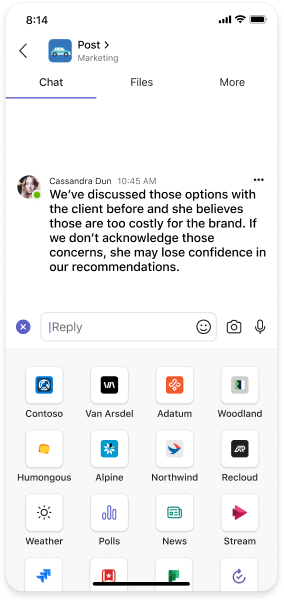This is a detailed description of a screenshot from a distorted mobile device screen:

---

The image is a screenshot from a mobile device that appears stretched horizontally, altering its usual dimensions. The screen is split into two background sections: the top half is white, and the bottom half is a very light gray. 

In the top left corner, "8:14" is prominently displayed in bold black font. The top right corner showcases typical mobile icons: signal bar, Wi-Fi, and battery charge indicators. 

The main content of the screen starts with the heading "Post and Marketing." Below it, "Post" is listed as a subheading with an associated right arrow and a blue square icon featuring a blue vehicle.

Beneath this, three headers are listed horizontally: "Chat," "Files," and "More," with "Chat" currently underlined, indicating it is the active section. 

The chat section displays a message thread from a user named Cassandra Dunn. At 10:45 AM, Cassandra Dunn, whose profile picture is shown in a circle to the left of her name, posted in bold: "We've discussed those options with a client before and she believes those are too costly for the brand. If we don't acknowledge those concerns, she may lose confidence in our recommendations." 

Below this message is a reply text box. Inside the box are the word "Reply," a blue cursor to the left, and a smiley face icon. To the left of the reply box, there is a blue circle with a white arrow, presumably to close the box. To the right, there are camera and microphone icons, possibly indicating options to upload images or record audio/voice-to-text inputs.

The bottom half of the screen, which has a pale gray background, is arranged in a grid of app icons, organized into four columns and four rows. The apps in the top row are labeled Contoso, Van Arsdale, Datum, and Woodland. The second row includes Humongous, Alpine, Northwind, and ReCloud. The third row contains Weather, Polls, News, and Stream. The fourth row is partially visible, with some labels out of view.

Overall, the screenshot captures a detailed display of a chat interface within a marketing tool, framed by typical mobile interface elements and additional app icons.